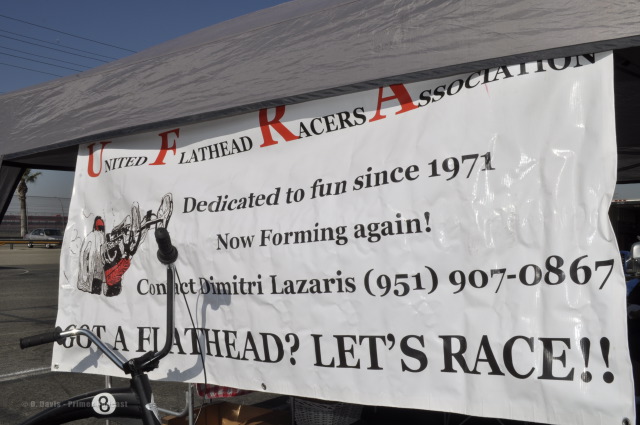The photograph, taken outdoors under a bright blue sky, showcases a white banner hanging from the awning of a gray tent. The banner prominently displays the title "United Flathead Racers Association" in large letters, with the initials 'U', 'F', 'R', and 'A' rendered in red while the rest of the text is in black. Below the title, in smaller black font, it reads "Dedicated to fun since 1971. Now forming again. Contact Dimitri Lazarus 951-907-0867." At the bottom of the banner, an emphatic message in uppercase black letters declares, "GOT A FLATHEAD? LET'S RACE." To the left of the banner, a black, chopper-style bicycle with black grips and an '8' ball design on its frame is parked, contributing to the nostalgic feel of the scene. The background includes elements of a typical outdoor setting with a clear sky, power lines, a parking lot, and a palm tree enhancing the vintage, community-oriented atmosphere of the image.